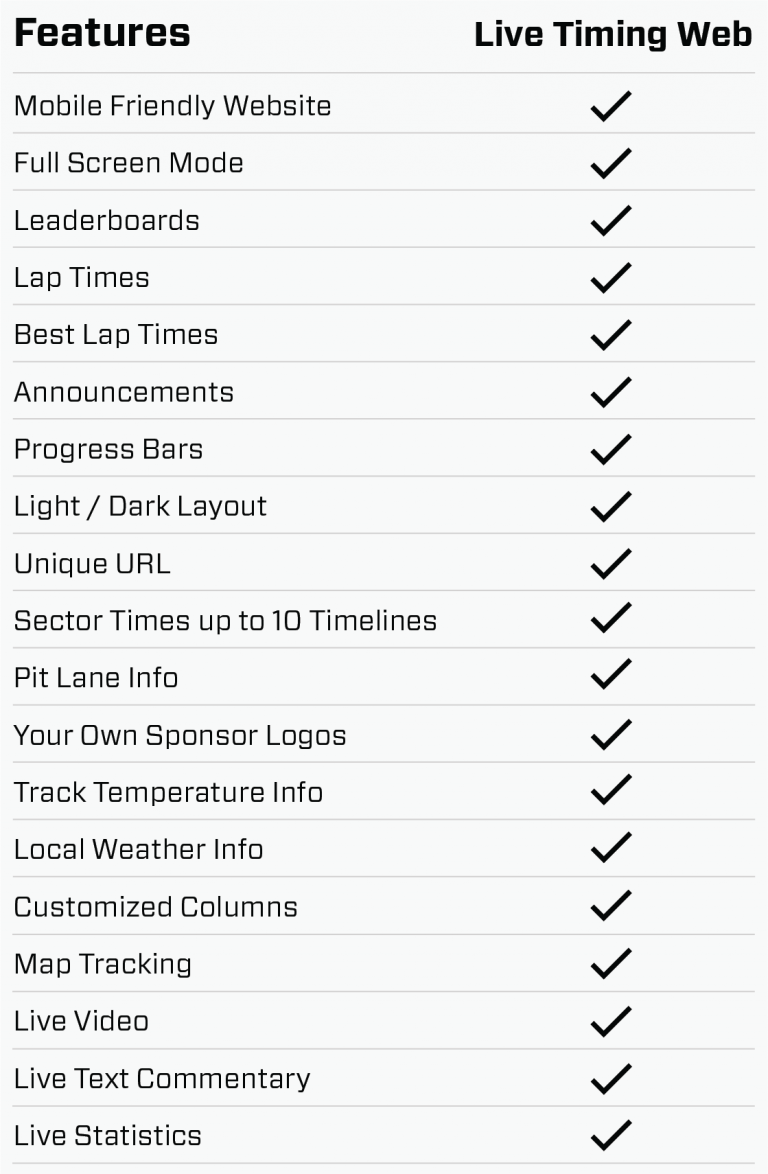This vertically oriented screenshot showcases a list of features for a "Live Timing Web" service, delineated by thin horizontal gray lines. The background is a very light gray and the text is displayed in a clear, readable format. At the top left corner of the image, the word "Features" is boldly highlighted in black. On the top right, "Live Timing Web" is similarly emphasized in bold black text. Each feature listed below "Live Timing Web" is marked with a prominent black checkmark, signifying its inclusion.

The features are itemized in regular black font and include the following, from top to bottom:

- Mobile Friendly Website
- Full Screen Mode
- Leaderboards
- Lap Times
- Best Lap Times
- Announcements
- Progress Bars
- Light / Dark Layout
- Unique URL
- Sector Times (up to 10 timelines)
- Pit Lane Info
- Your Own Sponsor Logos
- Track Temperature Info
- Local Weather Info
- Customized Columns
- Map Tracking
- Live Video
- Live Text Commentary
- Live Statistics 

Each feature is clearly separated by a thin gray line, ensuring a neat and organized presentation. This detailed enumeration highlights the inclusiveness and user-friendly aspects of the "Live Timing Web" service, emphasizing both its comprehensive data capabilities and customization options.